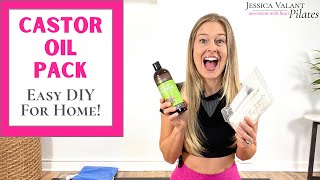The advertisement poster features a vibrant promotion for a Castor Oil Pack. In the forefront stands a blonde woman, mouth agape in excitement, holding a brown bottle with a green label in one hand and a white object in the other. She is dressed in a black crop top and pink pants, seemingly posing in a yoga studio adorned with white walls and a blue yoga mat to the left. Behind her, a small stool with a potted plant is barely visible. Prominent on the poster is a rectangular inset with a pink border, where bold pink text reads "Castor Oil Pack" and black text below announces "EZDIY for Home." To the right of the image, additional text states "Jessica Valens Pilates," emphasizing the promotional nature of the image. The overall setting and design suggest a targeted advertisement focusing on wellness and easy at-home DIY solutions.